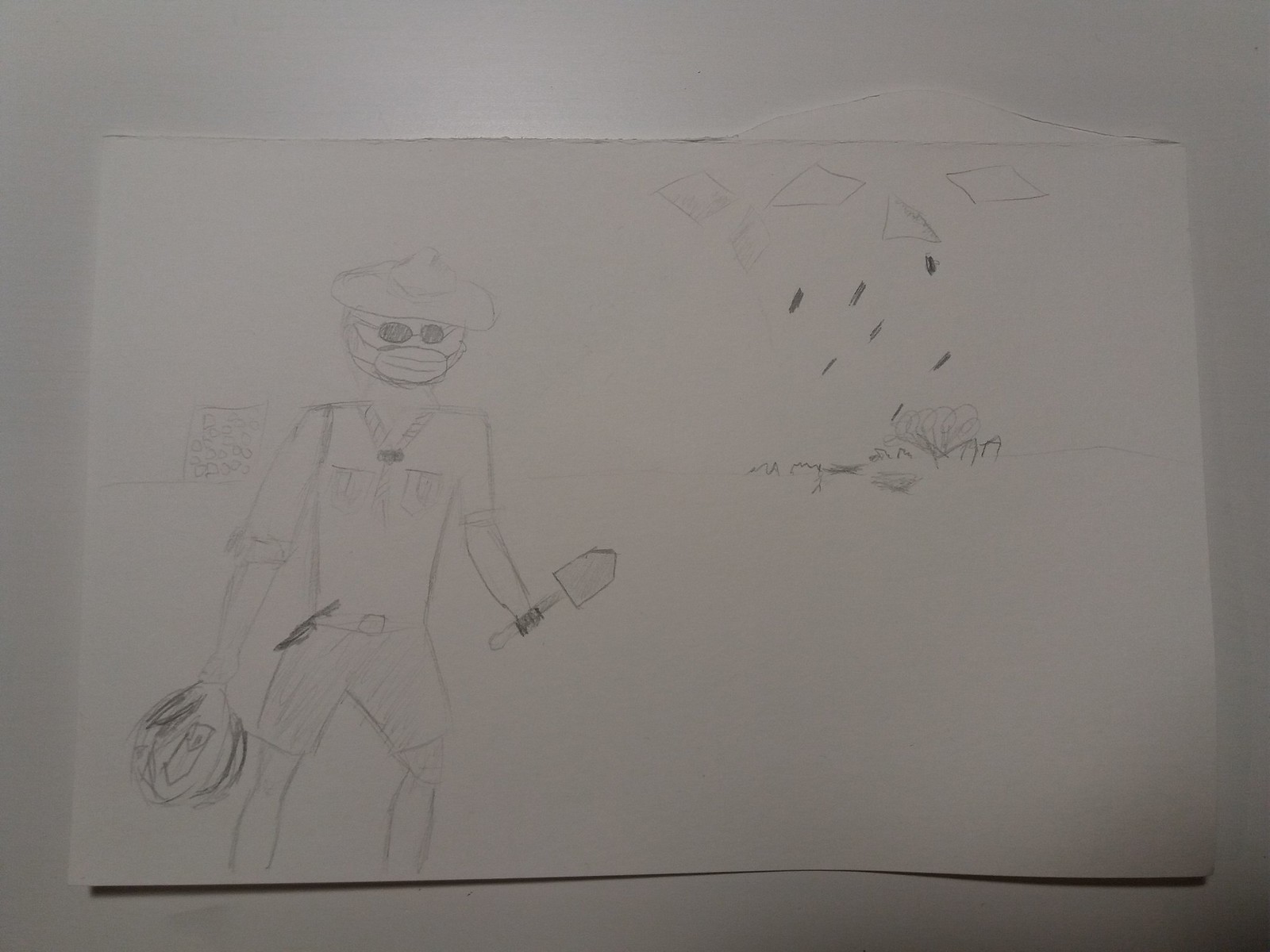A detailed pencil sketch rendered on light gray paper depicts an amateur drawing of a man standing against a plain background. The man, positioned mostly on the left side of the canvas, is characterized by his distinctive attire, including dark sunglasses and a dust mask covering his mouth. Atop his head sits a unique beret-style hat that resembles the top of an acorn. He is dressed in rolled-up sleeves, a white t-shirt with some writing on it, and white pants secured with a belt. In his right hand, he holds a small planter's spade, suggesting an intent to work in gardening. His frog-like head adds a quirky touch to the illustration. In the background, faint lines imply the falling of raindrops over a misty garden area where a spider is subtly drawn. The overall composition rests on a white surface devoid of color, enhancing the stark simplicity of this basic yet evocative sketch.